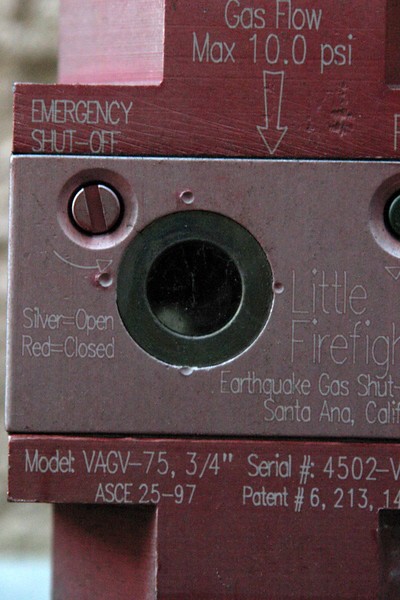This image presents a close-up, detailed view of what appears to be an old metallic earthquake gas shutoff valve, heavily labeled and adorned with various etchings and signs. Dominating the image is a device known as "Little Firefighter," as indicated by partial etching to the right of a central hole. The device is designed for emergency situations, with labels specifying its utility for earthquake gas shutoff, hailing from Santa Ana, California.

The central part of the image features a metallic plate with clear, thin-print lettering. At the top of this plate, an arrow points downward towards an "emergency shutoff" button. Below, the plate provides further instructions: "silver equals open," and "red equals closed." Additional text specifies the operational limits, including "max 10.0 PSI." The colors depicted are predominantly maroon at the top and bottom sections, with the middle showcasing various shades of gray and silver. 

Etched into the metal are also the model and serial numbers, partially visible as "model: VAGV-75, 3/4 inch, serial number: 4502-V." The truncated details continue with "A.S.C.E. 25-97" and a partially visible "patent number: 6,213,14..." Due to the tight zoom, the background is indistinct, with the image framed well enough to suggest it was taken outdoors, likely in broad daylight. This precise documentation hints at the aged yet crucial nature of the apparatus, underscoring its function in emergency gas flow control during seismic events.